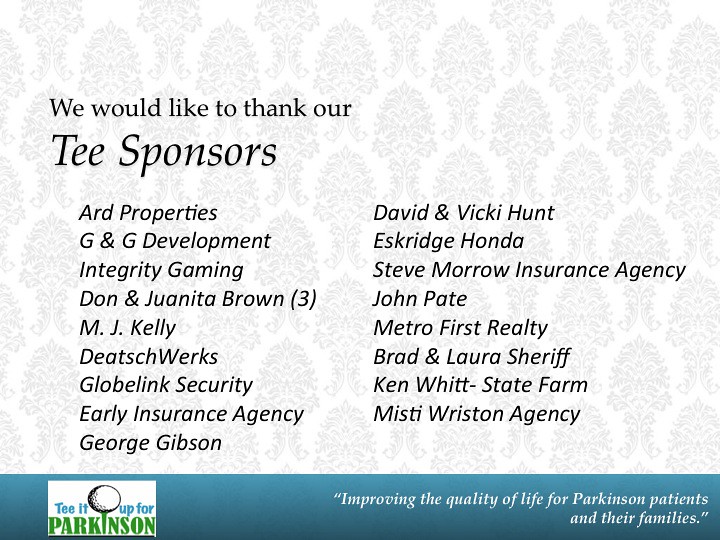This image appears to be a thank-you slide for sponsors, featuring text set against a white background with a subtle gray pattern. At the top, the black text reads: "We would like to thank our T sponsors." Below this heading is a comprehensive list of sponsors, which includes:

- ARD Properties
- G&G Development
- Integrity Gaming
- Dawn & Joannita Brown
- M.J. Catty
- Deitch Works
- Globelink Security
- Early Insurance Agency
- George Gibson
- David & Vicky Hunt
- Eskridge Honda
- Steve Morrow Insurance Agency
- Joan Pate
- Metro First Realty
- Brad & Laura Sheriff
- Kenwit-State Farm
- Misty Wriston Agency

At the bottom of the image, there is a blue horizontal strip. On the right side of this strip, more text states: "Tee it up for Parkinson's, improving the quality of life for Parkinson's patients and their families." Alongside this on the left side, there is an accompanying logo.